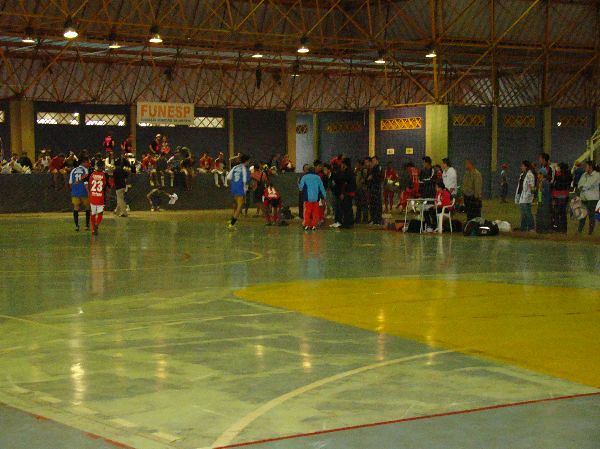In this indoor gymnasium with a tall, metal roof and exposed wood beams, we are on a court that appears to be designed for multiple sports. The court is primarily light blue with a brown section, and it features white lines for basketball, including the three-point arc and center court circle, as well as yellow markings for the free throw lane, and a red outline around the perimeter. Though the setting resembles a basketball court, the presence of players in blue and red team uniforms, including shorts and socks, suggests they might be engaged in an indoor soccer game or another type of sport—not basketball or volleyball as there are no nets or balls in sight. The gymnasium’s walls have a playful design, with a half-wall painted blue where some spectators are seated. The far background is filled with numerous people, some standing and others seated, all watching the event unfold. A prominent white banner sign with the text 'FUNE SP' hangs above the crowd, further adding to the bustling atmosphere of this indoor sports event.